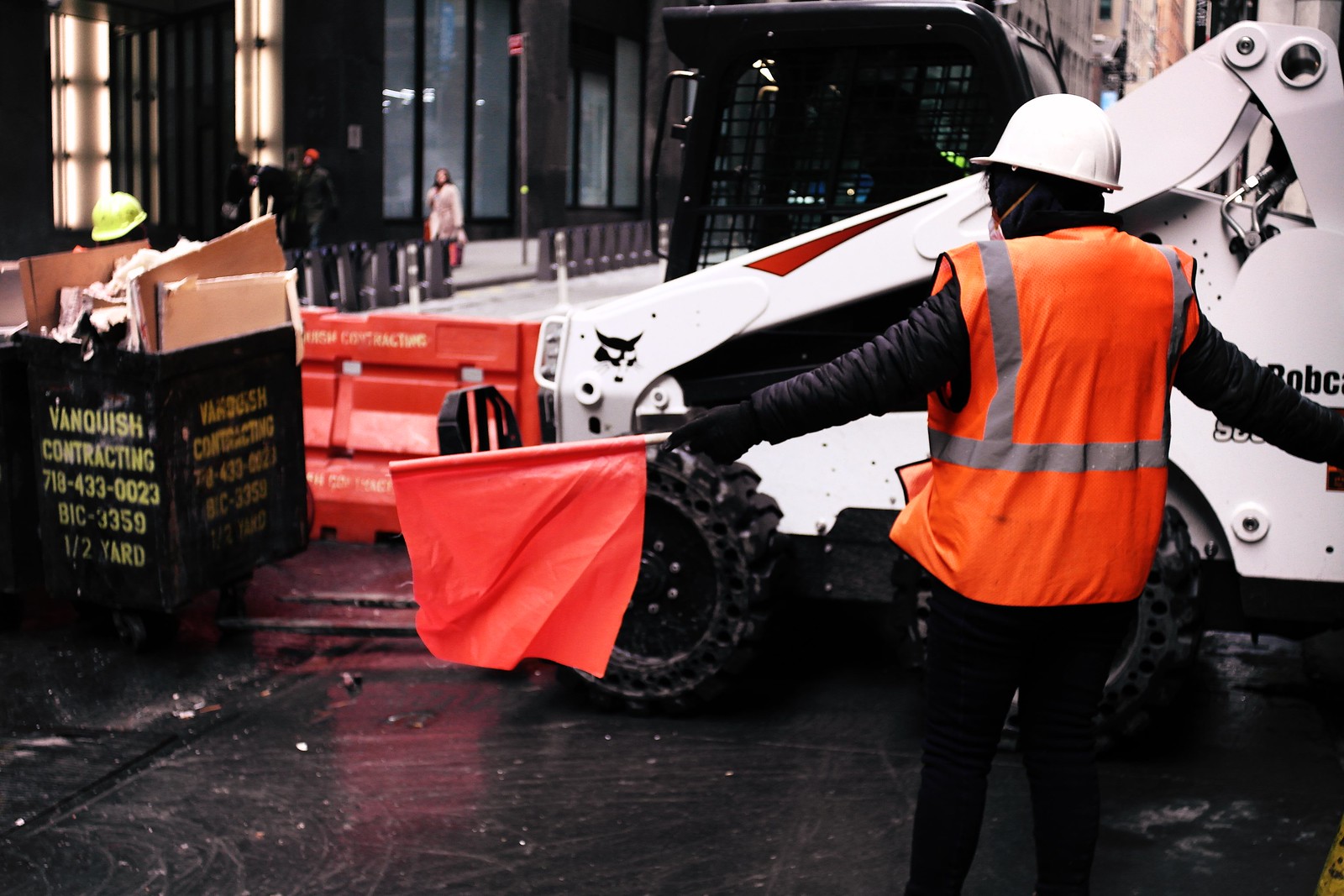This photo captures a bustling construction site situated in a busy city center. At the center of the image stands a construction worker in an orange vest and white hard hat, prominently holding a red flag to direct a large vehicle that appears poised to move a bin of construction waste materials. Adjacent to the worker is a red barrier wall, designed to protect pedestrians from the ongoing construction activities. The ground beneath is a smooth, solid black surface, and a basket containing folded cardboard boxes can be seen to the left. In the background, imposing buildings with tall glass windows and people walking around add to the urban atmosphere. The image is a vivid tapestry of colors, featuring shades of black, yellow, red, orange, gray, tan, white, and silver. The scene is set outdoors in the middle of the day, highlighting a dynamic moment within the construction zone.